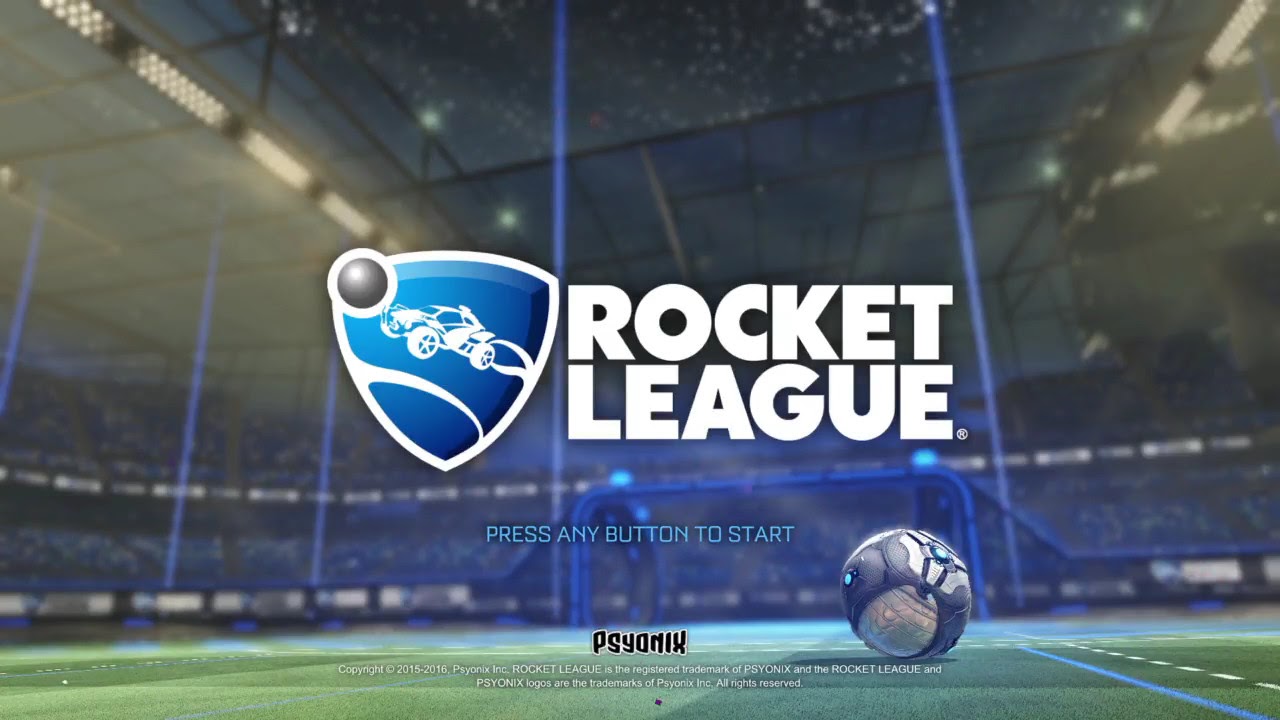This image is a detailed screenshot from the title screen of the video game Rocket League. Dominating the center a bit towards the left is a blue triangular shield outlined in white, featuring a white stylized car ascending from the lower left to the upper right. Inside the shield’s upper left corner is a gray circle also outlined in white. To its right, in bold white block letters, is the game's title "Rocket League." Below this, in smaller light blue text, it instructs "Press Any Button to Start," and underneath, the developer's name "Psyonix" appears in black with a white outline. The background of the image depicts the blurred interior of a grand stadium glowing with blue lights and surrounded by blue nets. On the green field at the lower right corner of the screen, a high-tech, gray and white soccer ball with blue electric detailing is positioned, emphasizing the game's futuristic soccer theme. The image is clearly marked with a copyright notice for the years 2015-2016 attributed to Psyonix.